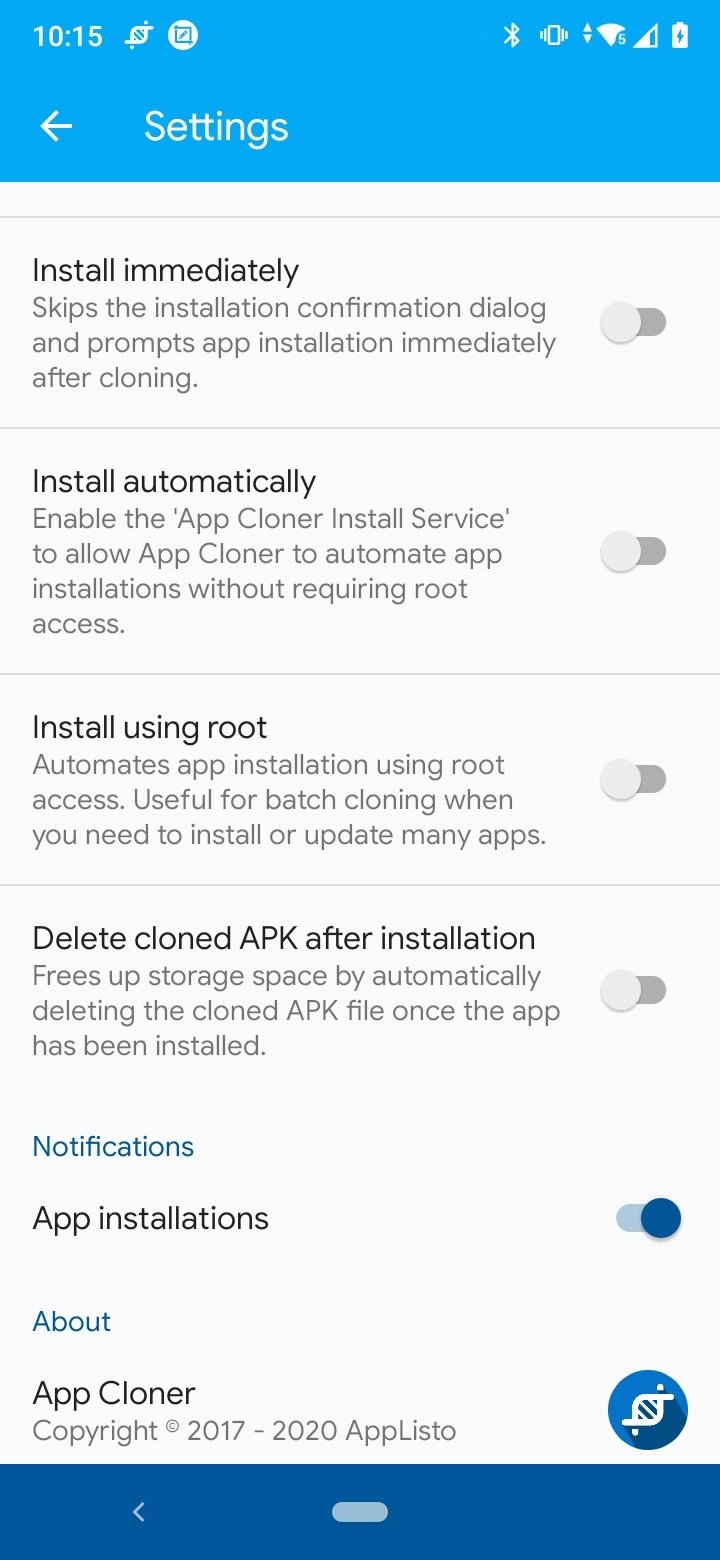**Screenshot Description:**

At the top of the screenshot, there is a light blue area displaying a status bar which includes the time "10:15", a Bluetooth icon, and a signal strength indicator showing 3 out of 5 bars. An arrow pointing left is also visible next to the word "settings."

Below the status bar, the screen shows a gray background with various installation options and descriptions. These options pertain to app installation settings, specifically for an app cloner. Each option has a toggle switch on the right side, all of which are gray and turned off. The options and their descriptions are as follows:

1. **Install Immediately**: "Confirmation dialog and prompts app installation immediately after cloning."
2. **Install Automatically**: "Enable the app cloner install service to allow app cloner to automate app installation without requiring root access."
3. **Install Using Root**: "Automates app installation using root access, useful for batch cloning when you need to install or update many apps."
4. **Delete Clone APK After Installation**: "Frees up storage space by automatically deleting the clone APK file once the app has been installed."

Each setting is displayed with a detailed explanation alongside a corresponding toggle switch for user interaction.